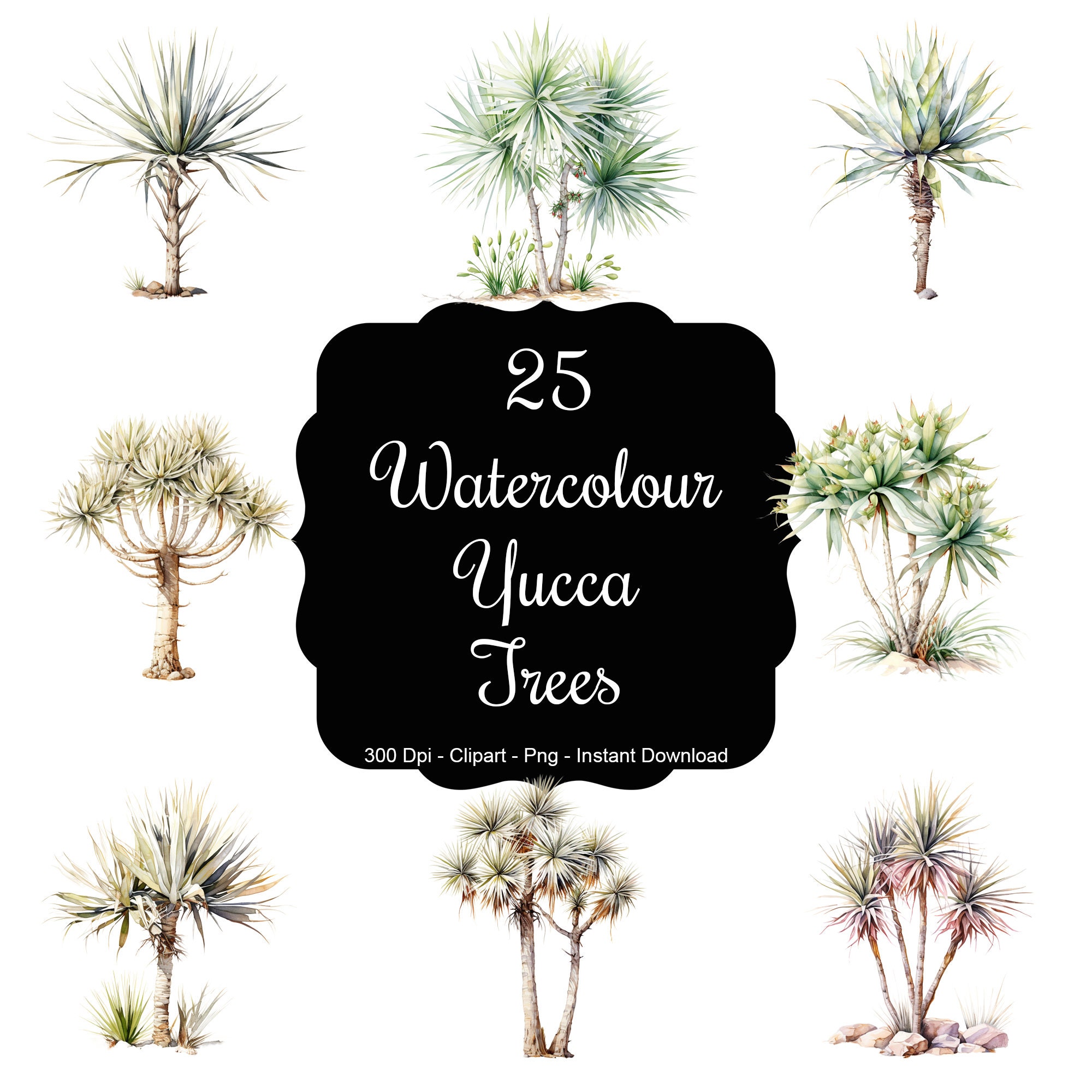The image is a promotional thumbnail for a set of 25 Watercolor Yucca Trees clip art available for instant download as PNG files at 300 DPI. Central to the design is a large, almost square, black sign featuring white, bouncy cursive text that reads "25 Watercolor Yucca Trees." Beneath this, smaller white text includes additional details: "300 DPI, Clip Art, PNG, Instant Download." Surrounding the sign are eight different watercolor illustrations of Yucca trees, with three positioned above, three below, one to the right, and one to the left. The trees are depicted in a variety of styles and colors, primarily greens but also featuring hints of pink, brown, yellow, and red. Each tree has distinctive sharp, protruding leaves, characteristic of the Yucca species, adding a touch of natural beauty to the advertisement.